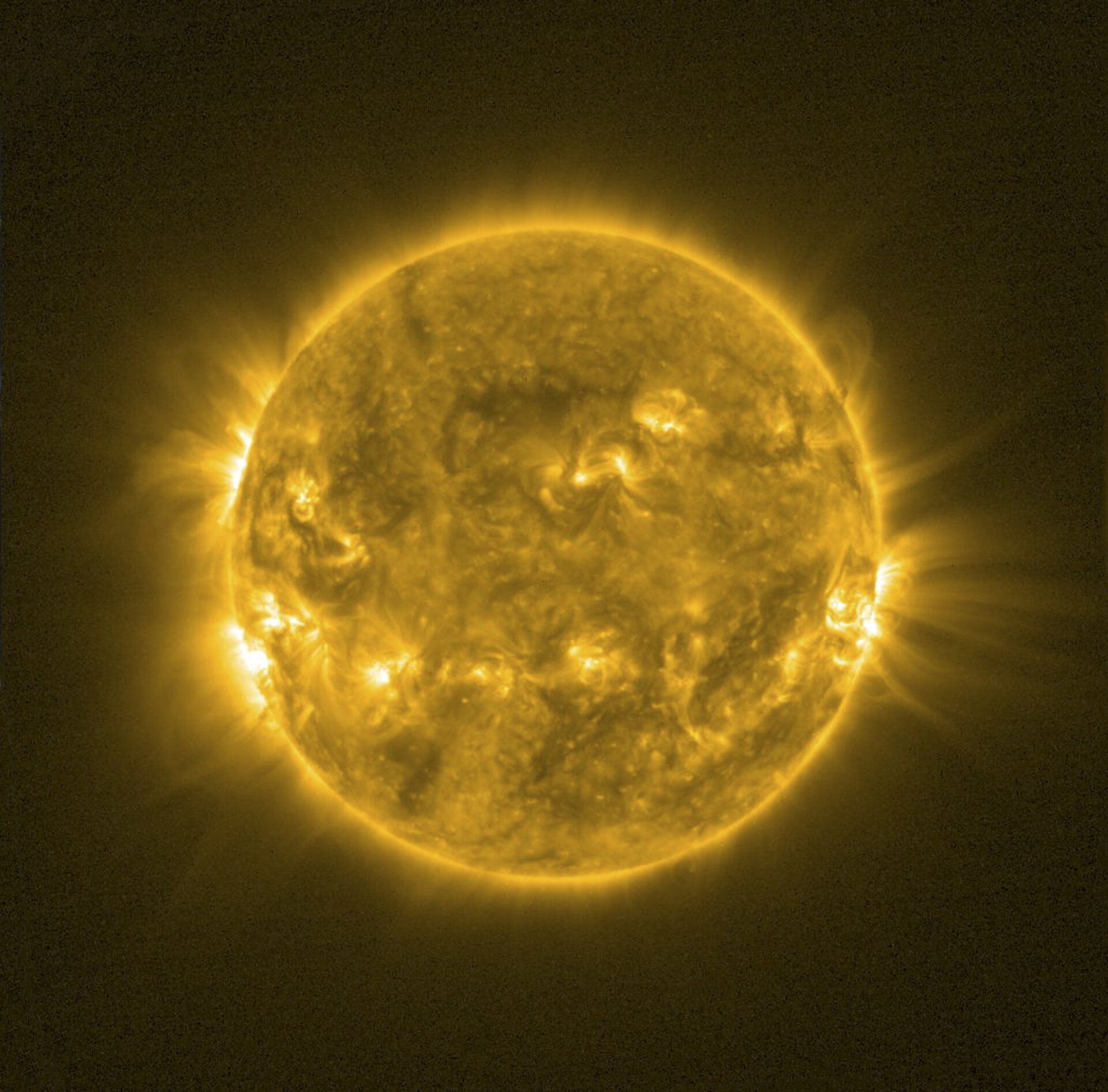This image, possibly a 3D render, showcases a striking depiction of the sun against a completely black background. The sun itself is presented as a brilliantly glowing yellow sphere, with several areas emitting a more intense yellow glow, likely representing sunspots. Around this solar orb, waves of gaseous eruptions can be seen flowing outward, adding dynamism to the scene. The dark background is textured with a subtle film grain, which does not affect the sun’s detailed and radiantly clear appearance at the center. This captivating image is solely focused on the sun, with no other celestial bodies or stars present in the frame, highlighting the sun's solitary grandeur.